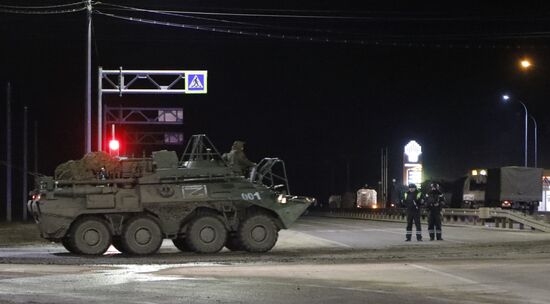This nighttime photograph captures a military scene, featuring a large, gray, eight-wheeled armored vehicle traversing a four-lane highway from left to right. The vehicle, possibly part of a convoy, is carrying undisclosed military equipment. In front of the vehicle stand two men, possibly Russian policemen, directing traffic. The men appear distant and their faces are indistinguishable, but they seem to be wearing coats. The scene is set in what looks like a business district or suburb, with several buildings lit in the background, including a prominently white-lit structure on the right side. Above the vehicle, there is a blue highway sign, and the photograph's upper edge shows some telephone wires. The surroundings are dimly illuminated by street lights on the right and left sides of the image.